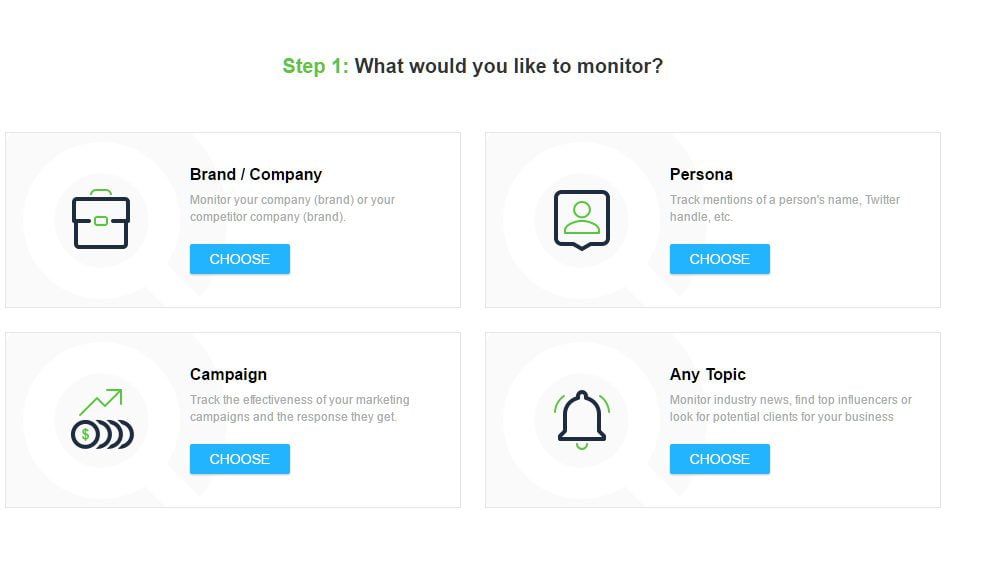The image features a clean, white background with the heading "Step 1" in green text at the top. Below this heading, the question "What would you like to monitor?" is displayed in black text. Four sections of information are presented, each within blue and white boxes outlined in light blue.

1. The first box has an icon of a briefcase and is labeled "Brand/Company." It explains, "Monitor your company brand, PR, or your competitor's company brand." Beneath this description is a blue button labeled "Choose."

2. The second box is labeled "Campaign." It outlines, "Track the effectiveness of your marketing campaigns and the response they get." This also includes a blue "Choose" button at the bottom.

3. The third box is titled "Persona." It states, "Track mentions of a person's name, Twitter handle, etc." and, like the others, contains a blue "Choose" button.

4. The fourth and final box is labeled "Any Topic." It offers the option to "Monitor industry news, find top influencers, or look for potential clients for your business." As with the other sections, it includes a blue "Choose" button.

Each section provides a clear and concise option for what users can monitor, helping them make an informed choice tailored to their needs.